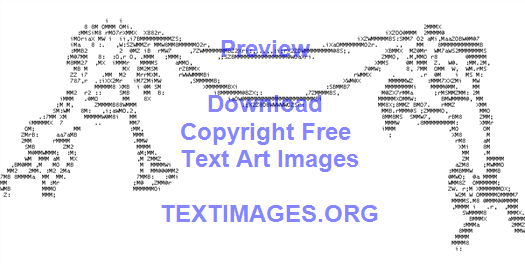The image features two characters holding up a banner with typed letters. The character on the left, who leans forward slightly, uses one hand to hold the bottom and the other to hold the top of the banner, with a tassel hanging from their top hand. The character on the right stands straighter, with thicker limbs, and holds something solid in one hand while using the other to support the banner. 

The banner has a distinctive shape, swooping down deeper at the bottom than at the top. The text on the banner is center-justified and in a light purplish color. It reads: "Preview" at the top, followed by "Download," "Copyright," "Free," "Text Art Images," and "textimages.org" at the bottom. Notably, there is a double space between "Preview" and "Download," as well as between "Text Art Images" and "textimages.org." The background of the image is completely white.

The drawing is an ASCII art representation, with one character resembling a flying cherub holding a trumpet, while the other figure appears to be a man with goat legs. The scene is designed to highlight the text, creating a visually engaging and whimsical promotion for the website textimages.org.